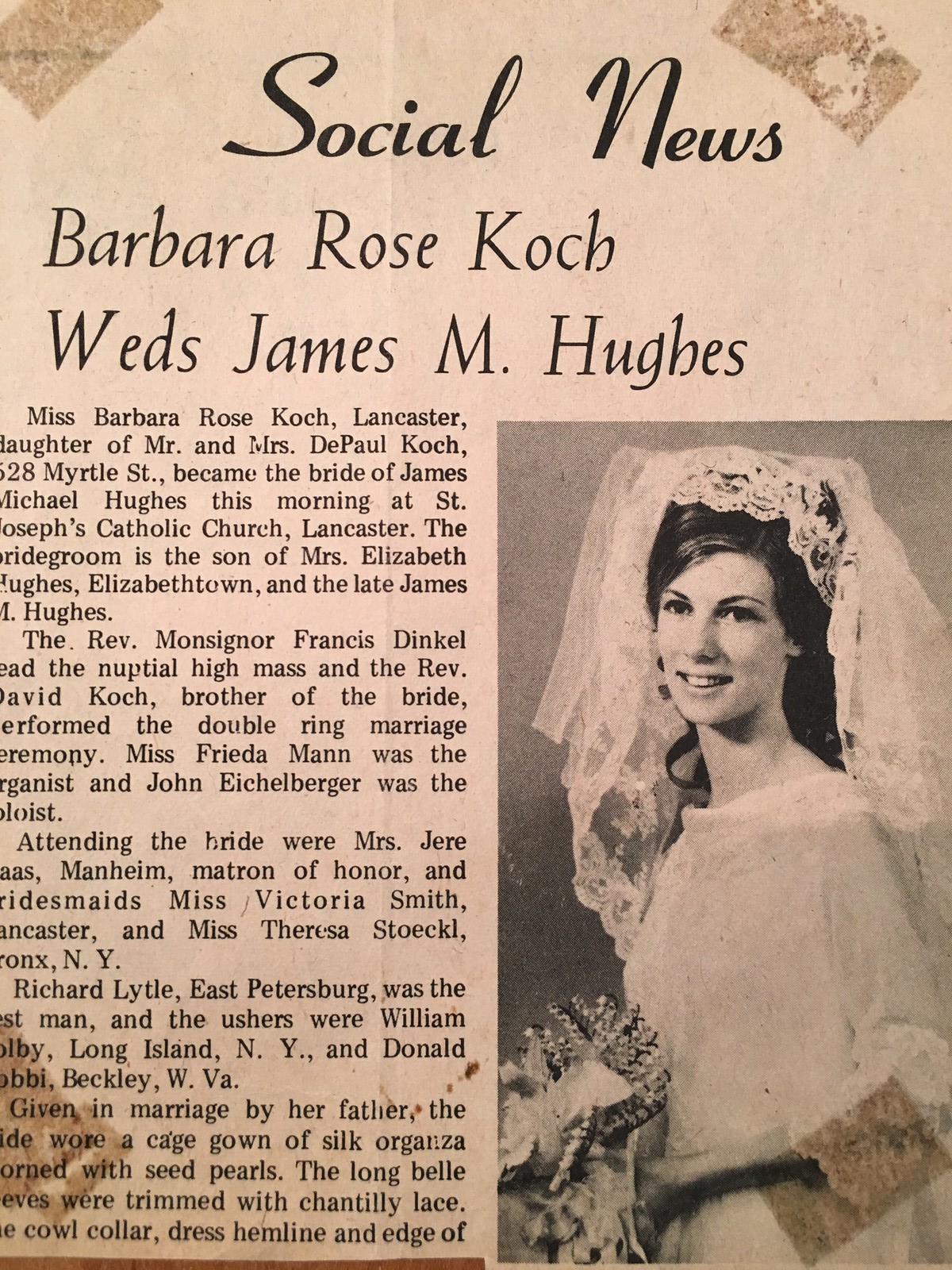The image depicts an old, faded newspaper clipping with a pinkish tint and tape marks at the corners, indicating it was once affixed to a scrapbook. The clipping is a social news announcement with a bold heading that reads, "Social News: Barbara Rose Koch weds James M. Hughes." The text is organized in columns, with the article on the left and a black-and-white photo on the right.

The photo features a slender, smiling bride in a white wedding dress adorned with a poofy lace headband veil, holding a bouquet in front of her while looking from right to left. The article announces, "Miss Barbara Rose Koch, Lancaster, daughter of Mr. and Mrs. DePaul Koch, 528 Myrtle Street, became the bride of James Michael Hughes this morning at St. Joseph's Catholic Church, Lancaster. The bridegroom is the son of Mrs. Elizabeth Hughes, Elizabethtown, and the late James M. Hughes."

The Reverend Monsignor Francis Dinkle officiated the nuptial high mass, and the Reverend David Koch, brother of the bride, performed the double ring ceremony. The clipping also mentions the organist Freda Mann and the soloist John Ehrlichman, along with additional details of the wedding further down the page.